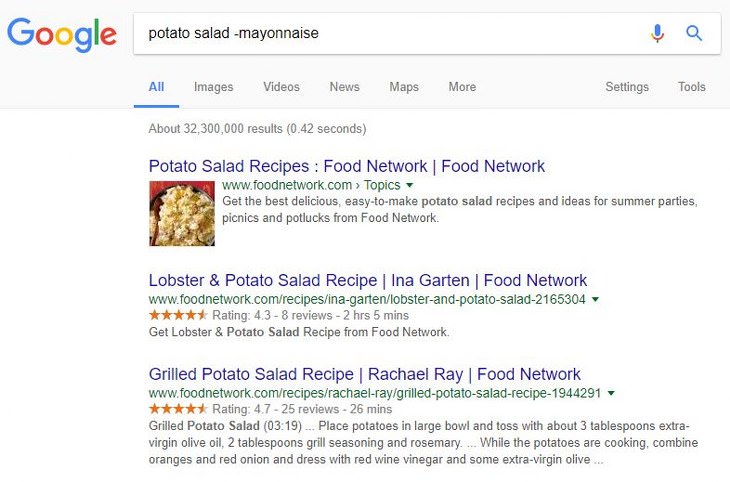The image displays a Google search result page featuring the Google logo on the left and the search bar to its right, with the query "potato salad and mayonnaise" entered. Below the search bar are various tabs including "All," "Images," "Videos," "News," "Maps," "More," "Settings," and "Tools." 

The search yielded approximately 32 million results in 0.42 seconds. The first result is a link to a "Potato Salad Recipe" from Food Network, including an image of potato salad. The URL displayed is www.foodnetwork.com, and it invites users to explore easy-to-make potato salad recipes and ideas for summer parties, picnics, and potlucks.

The second result is for a "Lobster and Potato Salad Recipe by Ina Garten," also from Food Network. The URL for this recipe is www.foodnetwork.com/recipe/ina-garten/lobster-and-potato-salad-2165304. This recipe has a rating of 4 out of 3 stars based on 8 reviews, and the preparation time listed is 2 hours and 5 minutes.